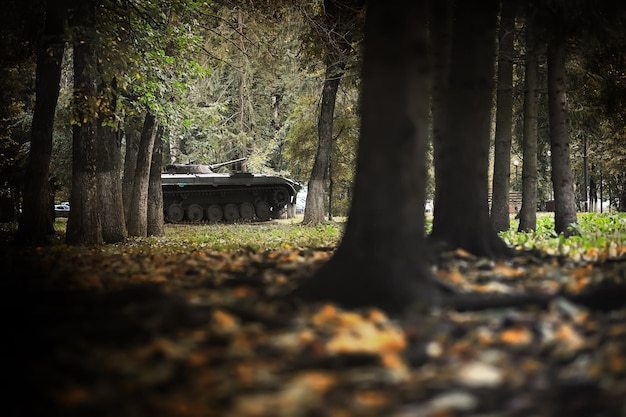In this color photograph, taken in a dense, gloomy forest during what appears to be autumn, the scene is both eerie and atmospheric. The forest floor is blanketed with fallen leaves, creating a natural carpet amidst the diverse array of tree trunks, some almost black and others showing white patches near the bottom. Light dapples in the foreground, capturing the essence of the season. Towards the background and partially obscured by the thick trees, there is a menacing military tank, suggesting a modern-day context rather than a historical one. The tank, gray and metallic, equipped with a prominent gun, appears to be advancing on a road. Its rollers are visible, indicating motion. This juxtaposition of dark, densely wooded areas in the foreground and the open, grassy area in the background adds a dramatic tension, evoking a feeling of dread as the viewer imagines the looming threat of the tank moving through the forest. The overall atmosphere of the photograph is one of foreboding, capturing the ominous presence of the tank against the serene but shaded woodland setting.